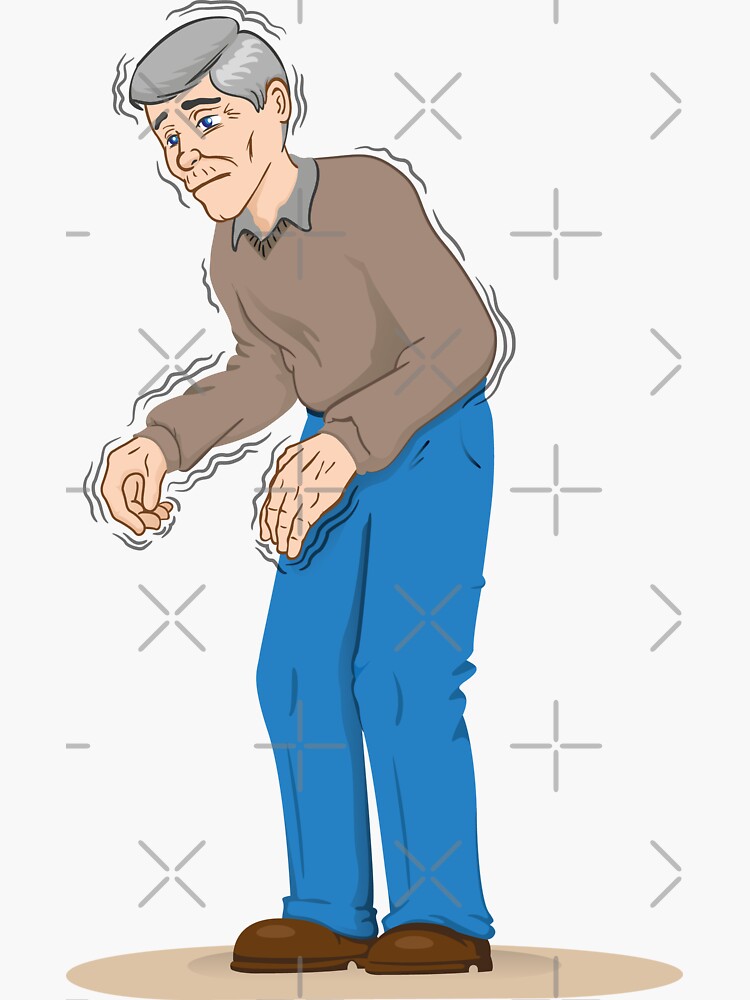The digital illustration depicts a very elderly man with short gray hair, fair skin, and blue eyes, facing towards the left. He is hunched over at the hip, with his arms held up uncomfortably, giving the impression of experiencing tremors or shakes. The man is dressed in a brown sweater over a gray shirt, blue pants, and brown shoes. He stands on a tan-colored circle or spot. His expression is sad and somber. The background is white with a pattern of light gray crosses and X's, adding a subtle texture to the image. Additionally, wiggly lines around his head, arms, and upper body visually emphasize the trembling or physical disturbance he is experiencing, giving the illustration a cartoony yet poignant look.